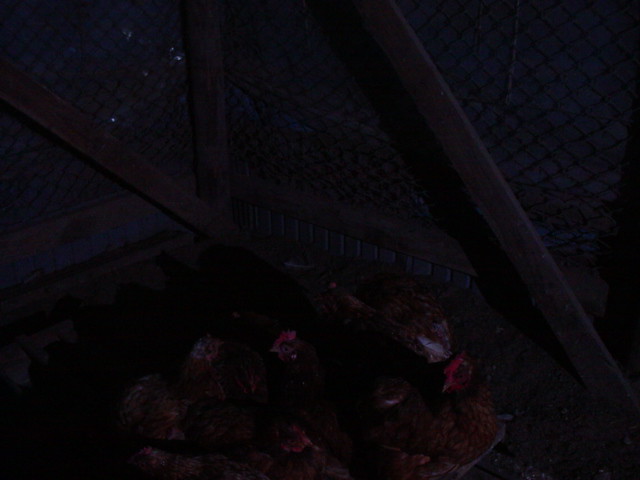In the dimly lit image, likely taken at nighttime, a small group of reddish-brown hens, numbering around five or six, are huddled together on the dirt floor of a chicken coop. Their bright red combs are faintly visible through the darkness, helping to identify them. The chicken coop itself is constructed with a wooden frame and reinforced by diagonal wood beams. It is enclosed with a chain-link screen. Behind the coop, there is a cinder block wall that partially blocks a view of what might be a blue tarp or container. The overall scene captures the hens nestled closely together in this rugged night-time setting.